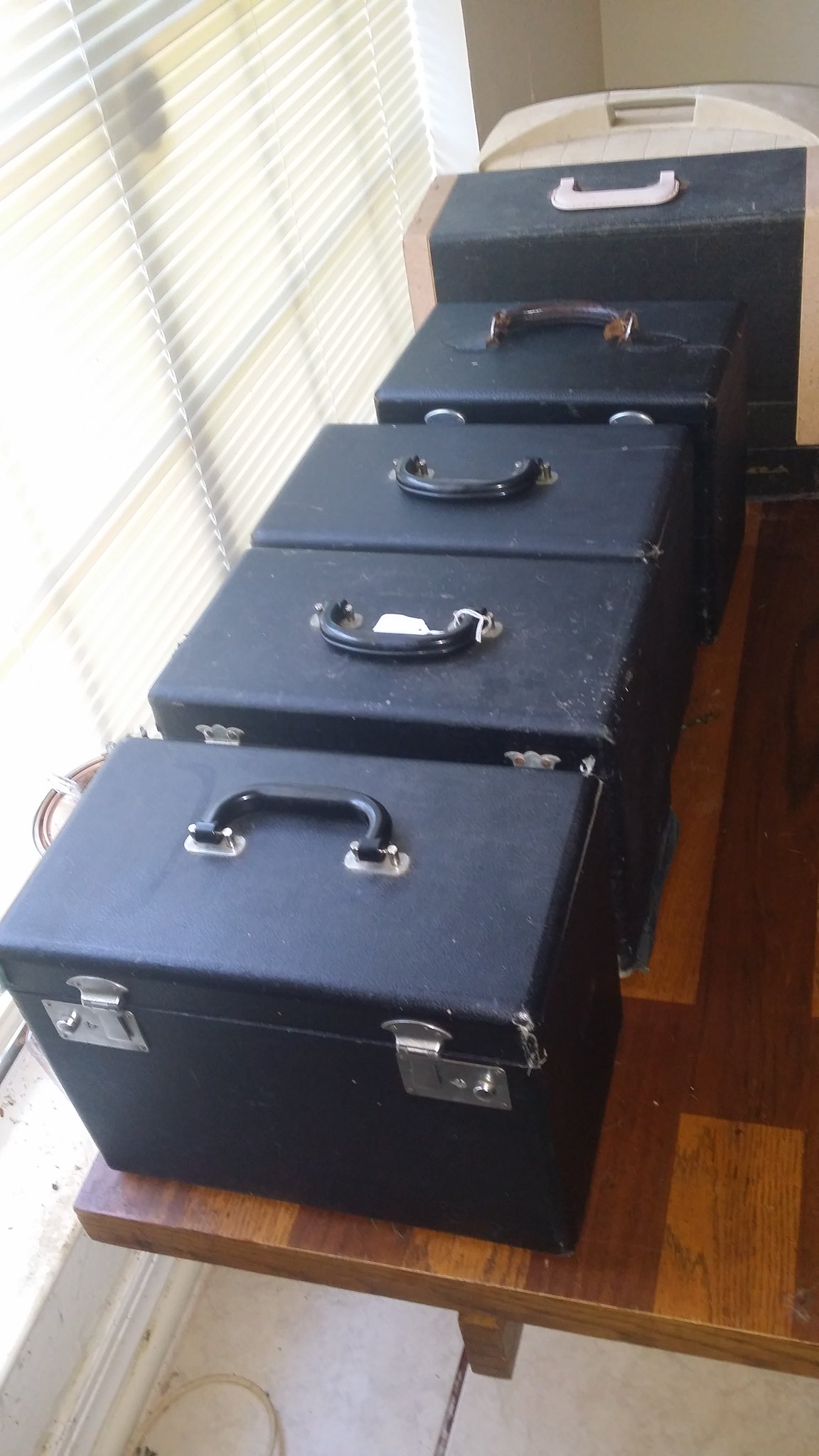The image captures a long, brown, wooden table with a distinct wood grain pattern, situated in a somewhat rough, homey setting with a tiled floor and a window to the left adorned with beige blinds. On the table rests a series of five old-fashioned, box-shaped briefcases, primarily navy blue with silver latches and hinges. Each has a handle on top, with the front three handles in black. Notably, the handle on the first briefcase is facing downwards. The second briefcase features a small white price tag tied around its handle. The fourth briefcase, contrasting the others, has a brown handle and appears worn. Further back on the table, there is a larger briefcase with white handles and beige edges. Behind this is another beige container with a built-in handle. The scene is bathed in daylight, suggesting a bright, sunny day outside.